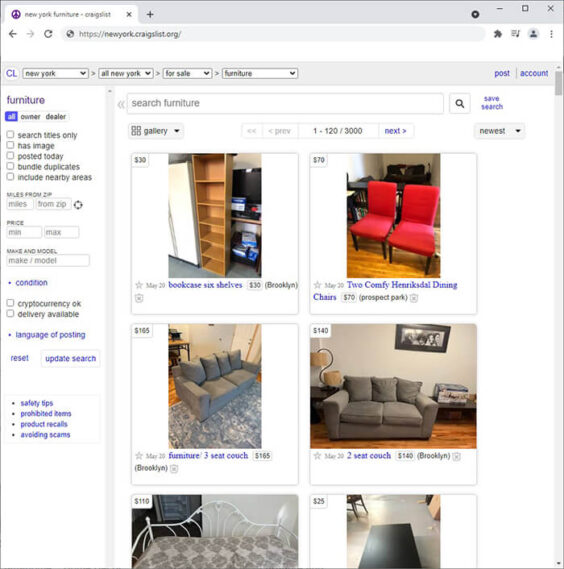Screenshot of a furniture sale webpage from New York Furniture Listings. The search query is "New York, All New York for sale, furniture," displaying a variety of second-hand items available for purchase. Listings include:

1. Six-shelf bookcase priced at $30.
2. Pair of Koofy Hinks dining chairs listed for $70.
3. Three-seat couch available for $165.
4. Two-seat couch priced at $140.
5. White-painted wrought iron day bed with a cushion for $110.
6. Dark-finished wooden table listed at $25. 

This detailed overview showcases various budget-friendly furniture options.